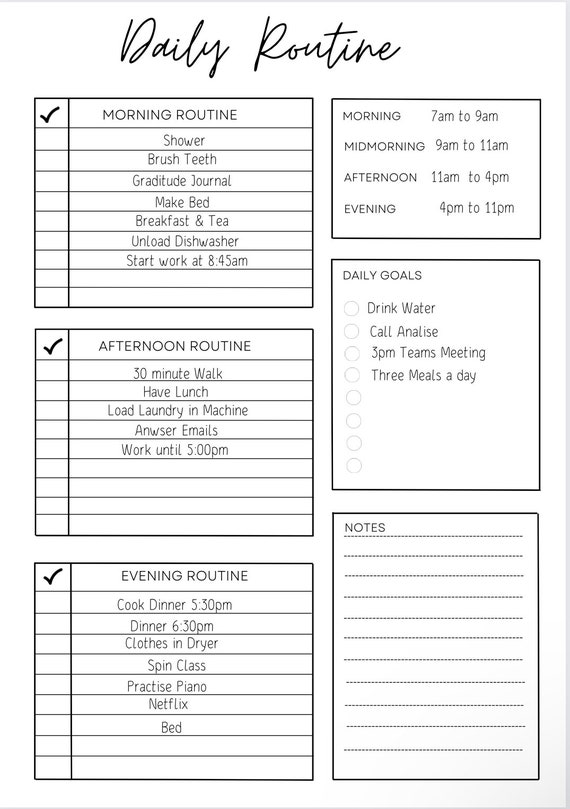The image displays a meticulously organized daily routine checklist on a white paper background, split into six distinct text boxes with checklists and time frames. The left side features a detailed schedule segregated into morning, afternoon, and evening routines, each with corresponding checkboxes.

- **Morning Routine (7 AM - 11 AM)**
  - Shower
  - Brush teeth
  - Gratitude journal
  - Make bed
  - Breakfast and tea
  - Unload dishwasher
  - Start work at 8:45 AM

- **Afternoon Routine (11 AM - 4 PM)**
  - 30-minute walk
  - Have lunch
  - Load laundry machine
  - Answer emails
  - Work until 5 PM

- **Evening Routine (4 PM - 11 PM)**
  - Cook dinner at 5:30 PM
  - Dinner at 6:30 PM
  - Transfer clothes to dryer
  - Spin class
  - Practice piano
  - Netflix
  - Bed

To the right of the paper is a structured grid detailing different time blocks:
- Morning: 7 AM - 9 AM
- Mid-morning: 9 AM - 11 AM
- Afternoon: 11 AM - 4 PM
- Evening: 4 PM - 11 PM

Additionally, there are two more text boxes on the right:
1. **Daily Goals**
   - Drink water
   - Call Annalise
   - 3 PM team meeting
   - Three meals a day

2. **Notes**
   - A blank space with black lines for personal notes

Overall, this image illustrates a comprehensive and organized schedule, highlighting essential daily routines, set goals, and time management for a structured day.